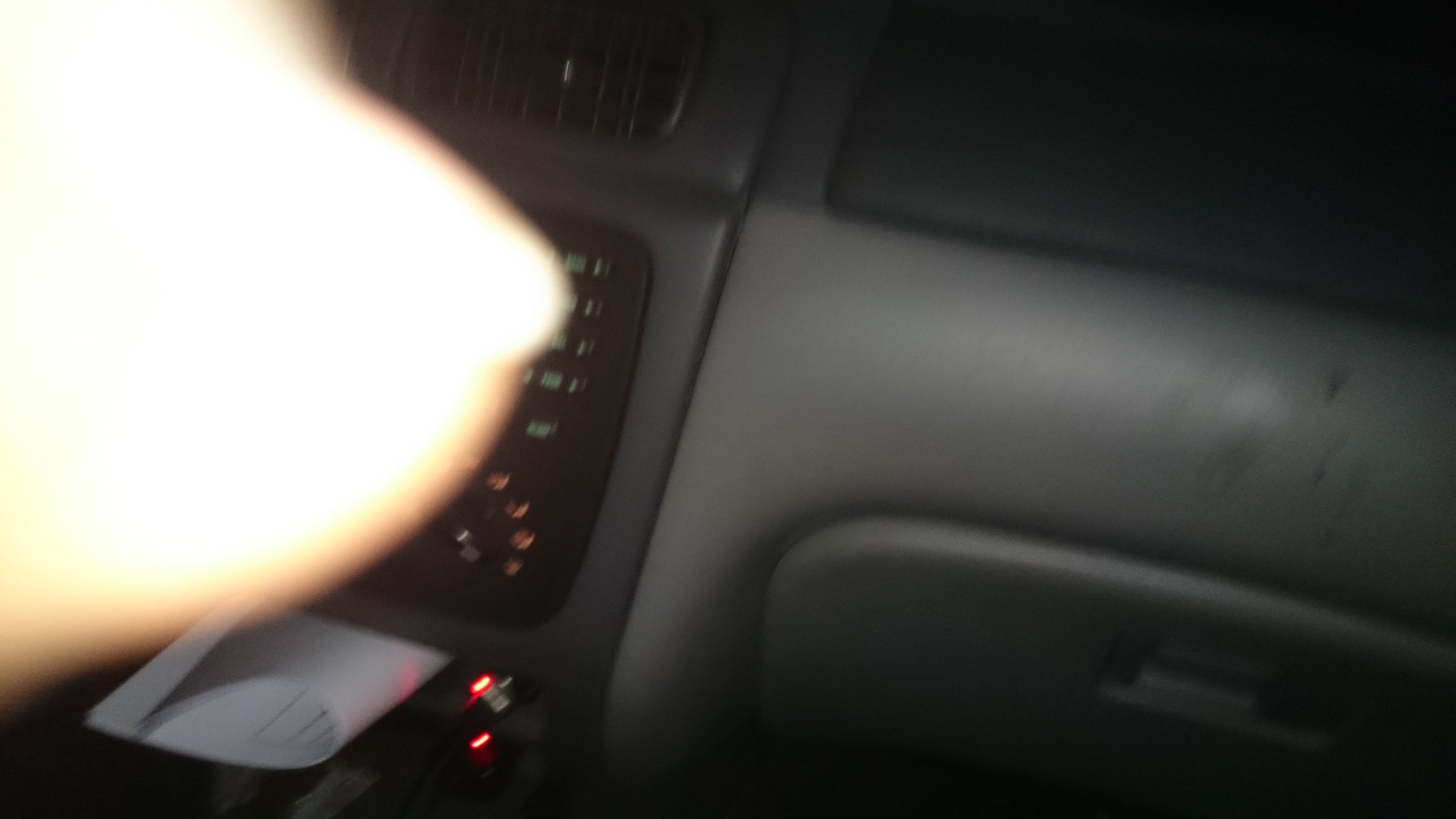A night-time view of a car dashboard, featuring the right side extending from the top of the dash down to part of the glove compartment, subtly illuminated by the vehicle's internal lighting. The image captures an array of controls and displays, though some are obscured by the photographer's index finger, partially extended with a slightly visible fingernail. Amidst the console clutter, there's a noticeable sheet of paper reflecting the dull red glow of illuminated messages and a few indicator lights at the bottom, possibly signaling warnings or inactive features.